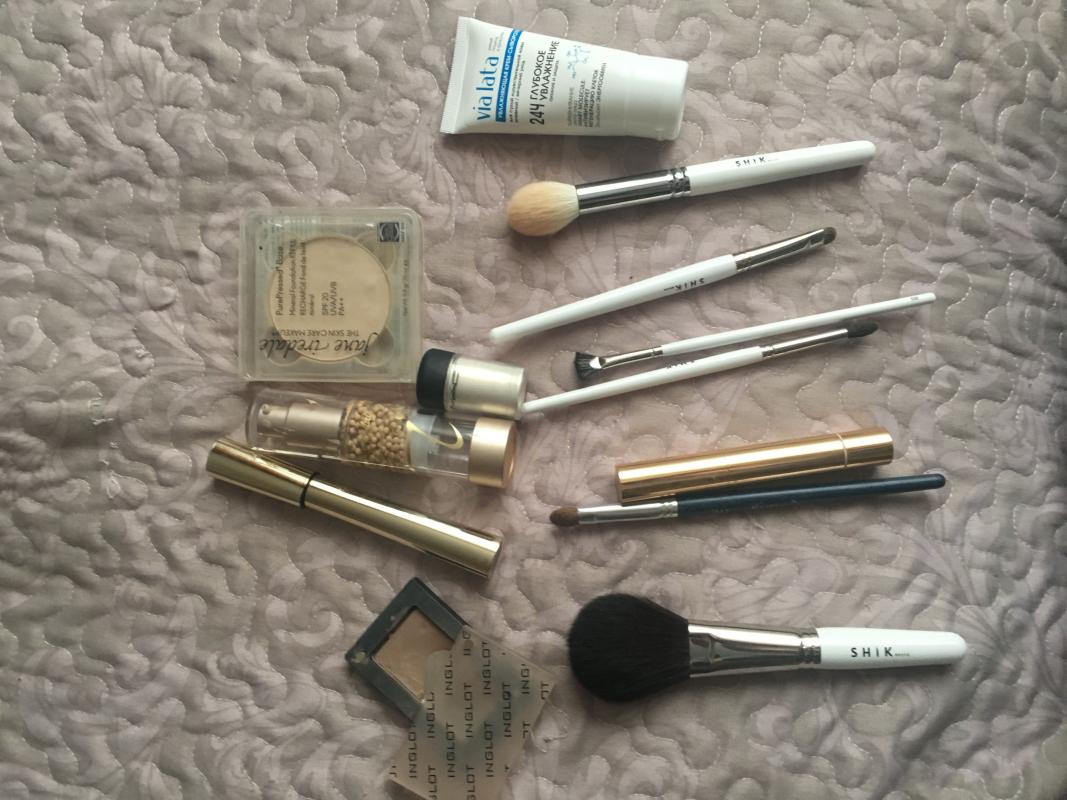In this detailed image, an assortment of makeup brushes and various cosmetics are meticulously arranged on what appears to be a quilted fabric, distinguished by its soft texture and subtle wavelike patterns.

On the left side of the image lies a compact of brown eyeshadow, positioned flat. Nearby sits a gold tube of mascara, identifiable by its lustrous exterior. Adjacent to these items is a clear spray bottle adorned with gold accents on its top and bottom, the specific function of which is unclear.

A small jar, associated with the brand MAC, might contain a form of powder makeup. Next to it, there is a typical circular compact, likely holding powder foundation. Moving to the right, a skincare cream container features the name "Violator" in blue print, though the smaller text is difficult to decipher.

Among the arrangement are several makeup brushes, varying in size and purpose. The moderate-sized brush, probably intended for cheeks or eyes, is followed by a smaller eye makeup brush meant for eyelid application. Another brush, more pen-like, is also present. The final item in the sequence is another gold-colored cosmetic product, next to which lies another small eyeshadow brush.

The last and largest makeup brush in the image, notable for its proportional handle to brush size, is likely designed for broader applications on the face, such as bronzer or foundation. This curated collection of beauty tools and products is elegantly displayed, each item thoughtfully placed on the textured fabric backdrop.